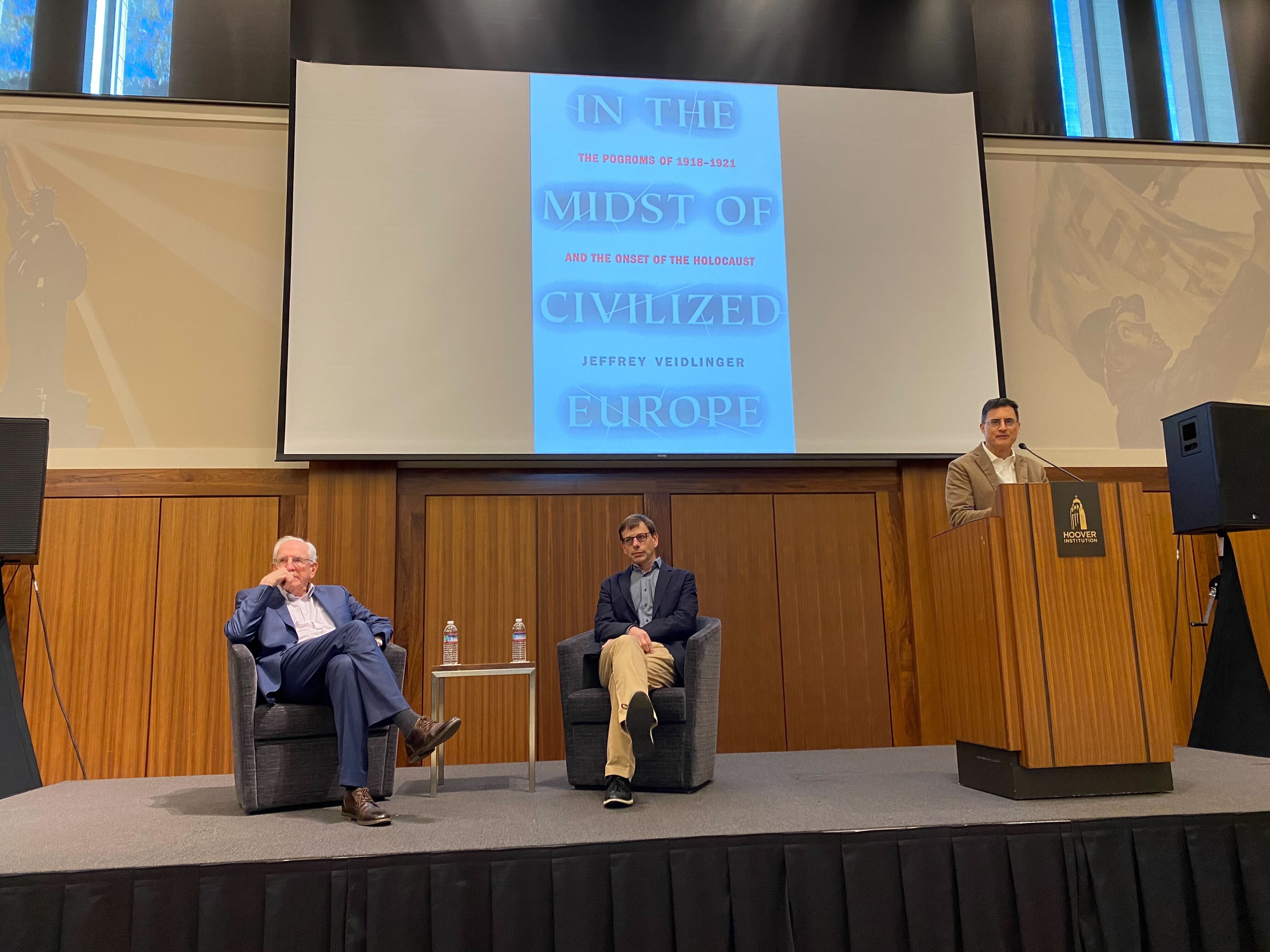This color photograph captures a conference presentation taking place on a stage platform, which features a light gray surface and black skirting around it. The platform hosts three men. On the right, a man stands behind a wooden podium bearing the label 'Hoover' and speaks into a microphone. He is dressed in a suit with a light brown jacket and glasses, looking directly at the camera. Flanking the podium are two dark gray chairs, each occupied by a man. The seated men, dressed in dark blue suit jackets, have their legs crossed; the man on the left is older and wears blue pants, while the man on the right dons yellow pants. Between these chairs is a small table with a water bottle at each end. Behind the trio is a large rectangular projection screen displaying the title of their talk: "In the Midst of Civilized Europe: The Pogroms of 1918 to 1921 and the Onset of the Holocaust," authored by Jeffrey Veidlinger. Additional smaller images, possibly depicting a soldier and the Statue of Liberty, are projected along the sides of the main screen. Light filters through tall windows partially covered by black curtains.